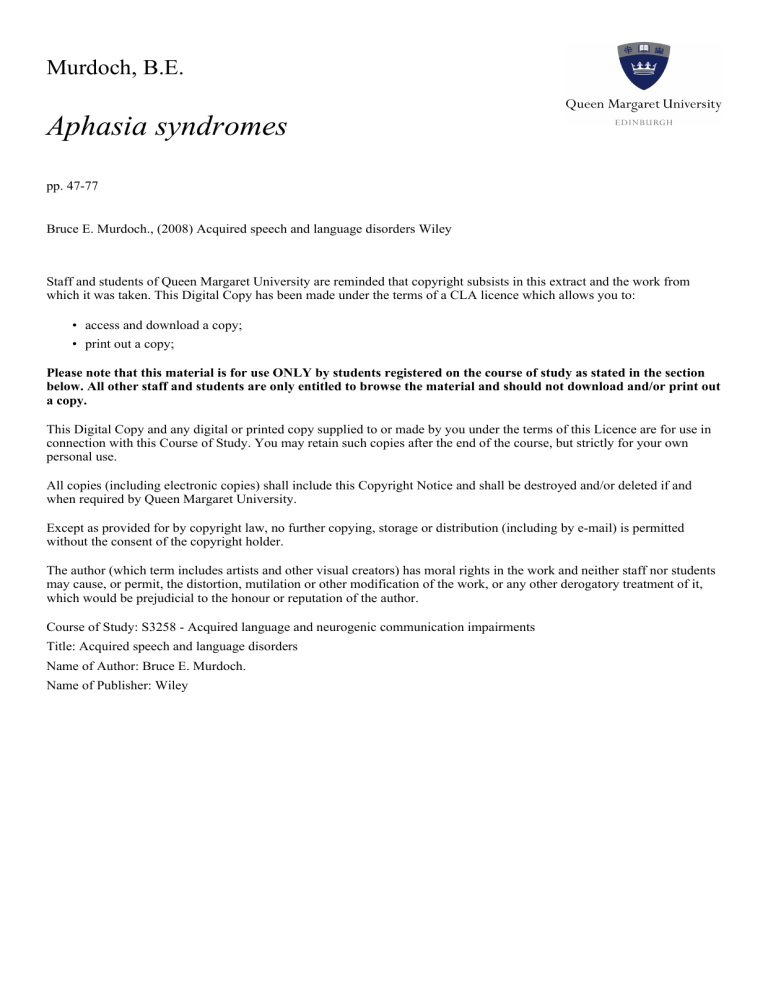This is a digital image featuring black text on a white background, detailing copyright and usage information for a particular academic resource. 

The top left of the image displays large black text that reads "Murdoch, B.E." with the letters "B" and "E" being capitalized and followed by periods. Below this, in an even larger italicized font, the text "Aphasia Syndromes" is prominently displayed. 

Following two line breaks, the next line in smaller black text reads "pp. 47–77". Underneath, after two more line breaks, there is a reference: "Bruce E. Murdoch (2008), Acquired Speech and Language Disorders, Wiley."

Three line breaks down, a paragraph of text reminds the staff and students of Queen Margaret University about the copyright associated with this extract, stating that it has been reproduced under the terms of a CLA license. The extract then details the permissions granted by this license with two indented bullet points:
- "access and download a copy;"
- "print out a copy;"

After another section break, there are three bolded lines emphasizing the restricted use of this material. The bolded text states that the material is for exclusive use by students registered in the specified course of study. It clarifies that other staff and students may only browse the material and are not permitted to download or print it.

Following an additional line break, the text continues in regular font, outlining the permissions related to this digital copy. It explains that copies made under this license are strictly for use in connection with the course of study and may be retained for personal use after the course concludes.